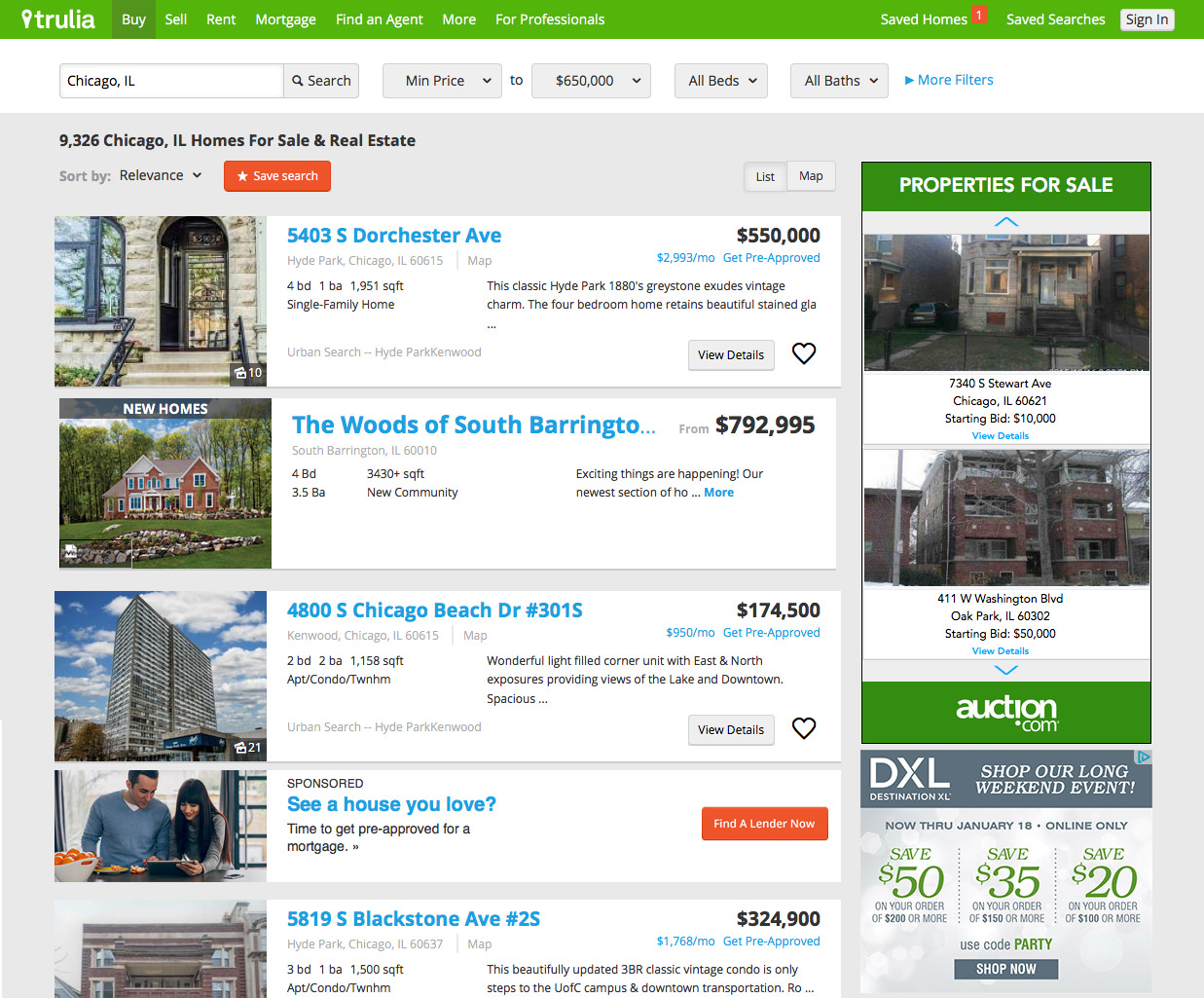A screenshot of the Trulia website showcases the top banner with the website's name, Trulia, and several navigation links: Buy, Sell, Rent, Mortgage, Find an Agent, More, and For Professionals. On the right side of the banner, options for Saved Homes, Saved Searches, and a Sign-In button are visible. Below the banner is the search information section, specifically displaying details for Chicago, Illinois. The search criteria include drop-down menus for minimum and maximum prices and options for "All Beds" and "All Baths," with an additional link for more filters to refine the search according to specific preferences.

The search results indicate that there are 9,326 homes for sale in Chicago within a maximum budget of $650,000, and all bed and bath options included. The results are currently sorted by relevance in a list format, though there is an option to view them on a map. Users can also save the search for future reference. 

The page displays four property listings:
1. A house on Dorchester Avenue with four bedrooms and one bathroom.
2. The Woods of South Barrington, the most expensive listing at $792,995, located in a new community.
3. A two-bedroom, two-bathroom apartment unit, which is a part of a condominium or townhome community.
4. A sponsored section featuring three additional homes.

Note: There was a mistake in the initial count; there are only three primary property listings shown before the sponsored section.